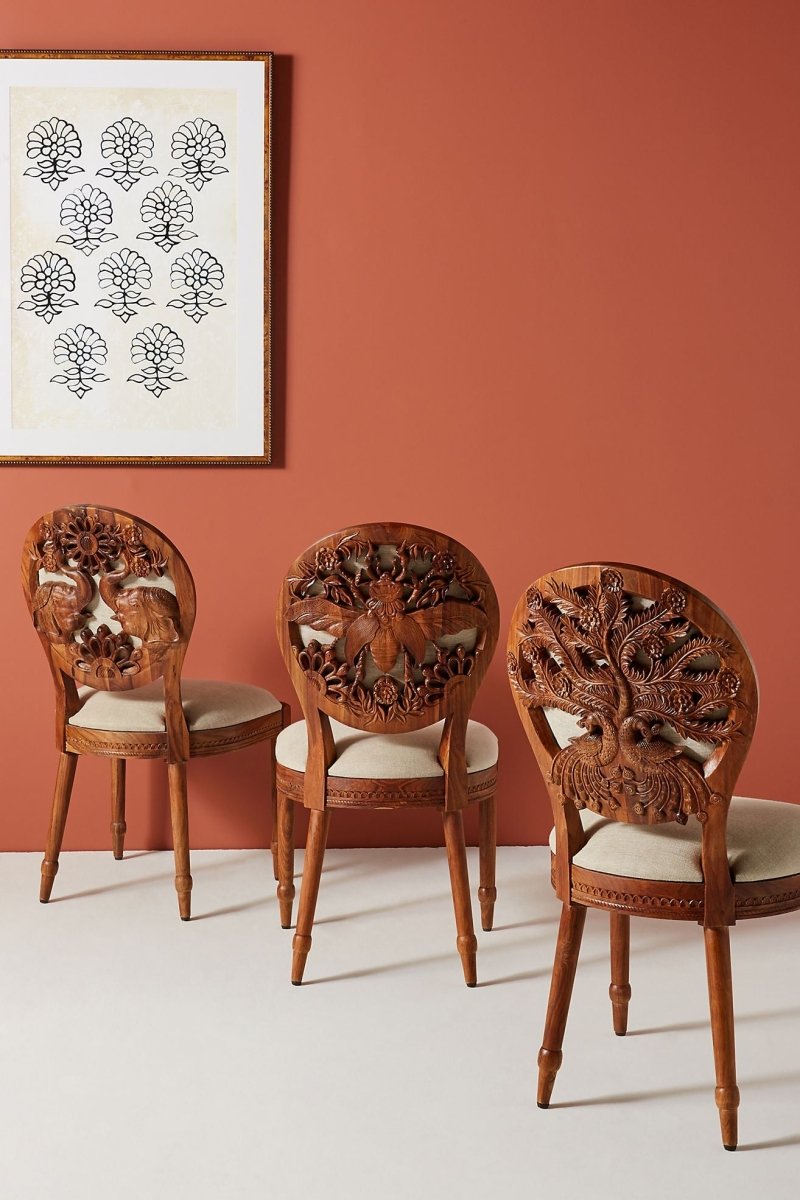This photograph depicts a tastefully decorated room, possibly a living or waiting area, featuring a white floor and a sand-colored wall that possesses an orangish-reddish-brown hue. Dominating the left side of the wall is a rectangular framed picture with a dark brown wooden frame. The artwork inside showcases a pattern of black or dark gray outlined flowers against a pristine white background, organized in a sequence of rows varying between three and two flowers each.
   
Three intricately carved wooden chairs are positioned diagonally from the bottom right towards the middle left of the image, their backs facing the viewer. The chairs, adorned with ornately detailed carvings, boast designs of a bird or bat, a bug or peacock, and two elephant heads. These chairs feature round seats covered in white fabric, supported by thin, spindly brown legs. The detailed engravings are a focal point, highlighting the craftsmanship and adding an artistic flair to the room's serene and elegant ambiance.